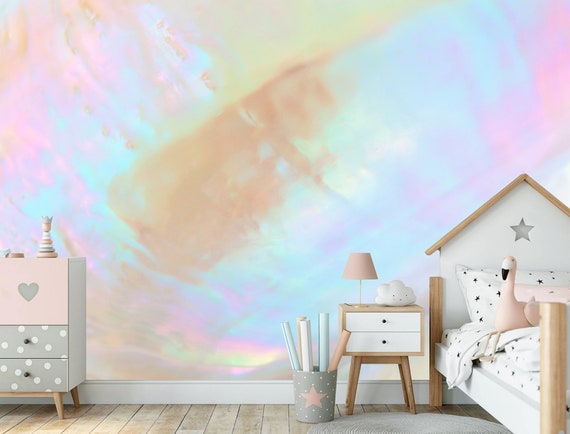The image depicts a children's bedroom with a charming mix of playful and cozy elements. On the far right side of the image is a low-standing single bed with a distinctive pitched headboard that is white, trimmed with natural wood at the top. The bed's frame, also white, features four natural wood posts. The bed is dressed in white sheets adorned with black stars and topped with a plush flamingo toy.

Adjacent to the bed is a nightstand with a European or IKEA-like design, characterized by wood trim and white drawers. On top of the nightstand sits a white cloud-shaped decoration and a peach-colored table lamp. Next to the nightstand, a grey trash can with white polka dots and a prominent pink star contains several tubes of wrapping paper.

A round, light grey rug is positioned near the bed, contrasting with the room's unfinished wooden floor. The room is bordered by a white baseboard. The left side of the room features a gray chest of drawers with white polka dots, and the upper compartment is pink with a grey heart. Decorative items rest on top of the chest, adding to the room's whimsical atmosphere. The room's walls are adorned with an iridescent, pastel rainbow pattern that gives a dreamy, almost photoshopped appearance.